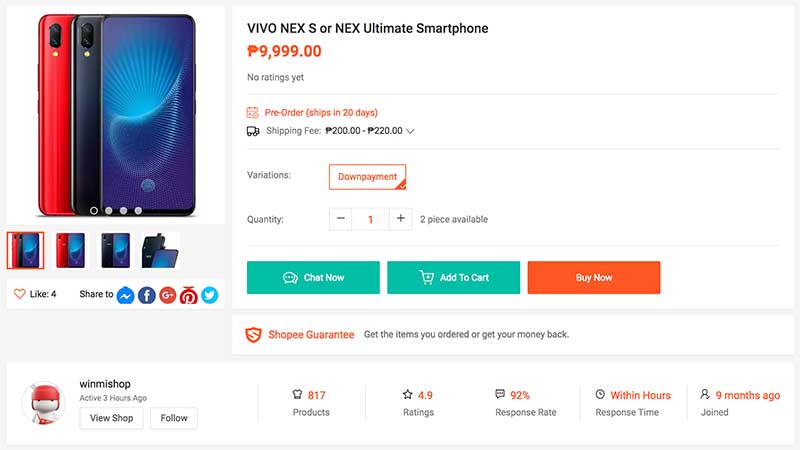The image showcases a section of a digital e-commerce website featuring smartphones for sale. Surrounding the main content is a gray border. On the left-hand side of the image, there are three smartphones displayed vertically: one red, one black, and one blue.

Beneath the smartphones, there are four smaller images showing different configurations of the devices. The listing has garnered four likes and offers sharing options to Facebook, Pinterest, and the now-defunct Google Plus, and Twitter.

On the right-hand side of the image, black text reads "Vivo Nex S" or "Nex Ultimate Smartphone." The price is displayed in a unique blue and orange dollar symbol format as $9,999.00. Underneath, gray text indicates "no rating yet" and mentions "pre-order ships within 20 days." There is also information about free shipping within a range of $200 to $220 in the mentioned dollar currency.

The listing includes options for down payment and quantity selection, showing that one or two pieces are available. Below these options are interactive buttons: two green buttons labeled "Chat Now" and "Add to Cart" in white text, and an orange button labeled "Buy It Now" in white text.

Additionally, there is a section featuring a seller profile, detailing ratings and response rates. It is noted that the seller joined the platform nine months ago.